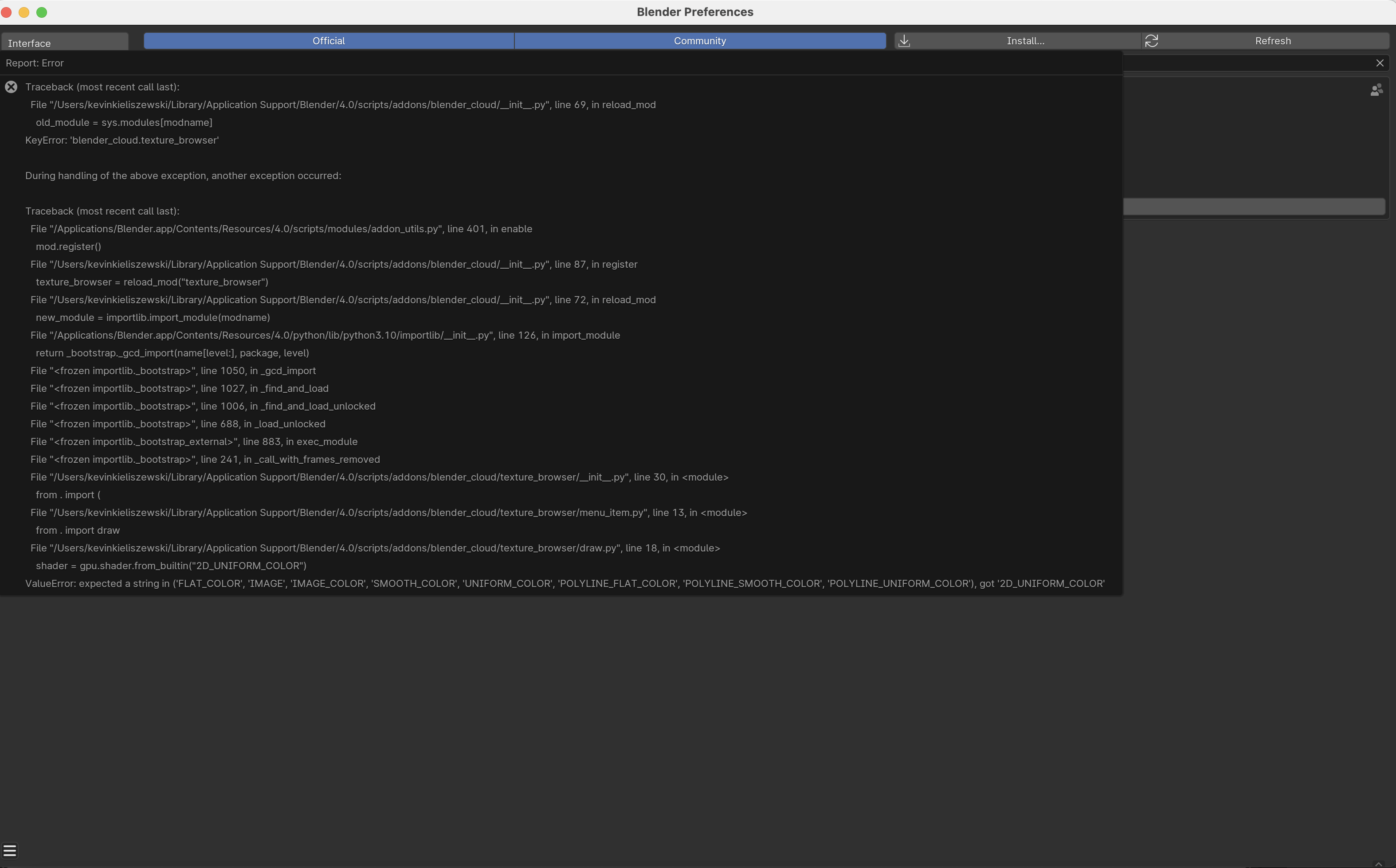The image depicts a screenshot of a black computer screen primarily filled with white text, indicative of a coding environment. At the top is a gray horizontal bar with the title "Blender Preferences" prominently displayed in the center. To the left of the title are three solid, filled-in circles colored red, yellow, and green respectively, possibly representing window control buttons.

Beneath this bar, the screen shows a section labeled "Interface" with a blue background that reads "Official Community". To the right of this, there are buttons labeled "Install" with a downward arrow and "Refresh" with two circular arrows pointing in opposite directions.

The remainder of the screen is dominated by a black background filled with a dense block of code. The code includes terms like "traceback", "most recent call last", and "file", followed by an extensive file name. Additionally, there is a mention of a "KeyError: blender_cloud.texture_browser" and a notice stating, "During handling of the above exception, another exception occurred."

This screenshot appears to capture the result of an attempt to compile or run a piece of code, which has resulted in an error message. The bottom of the screen contains further details about file locations and file names, indicating where the errors occurred within the codebase.